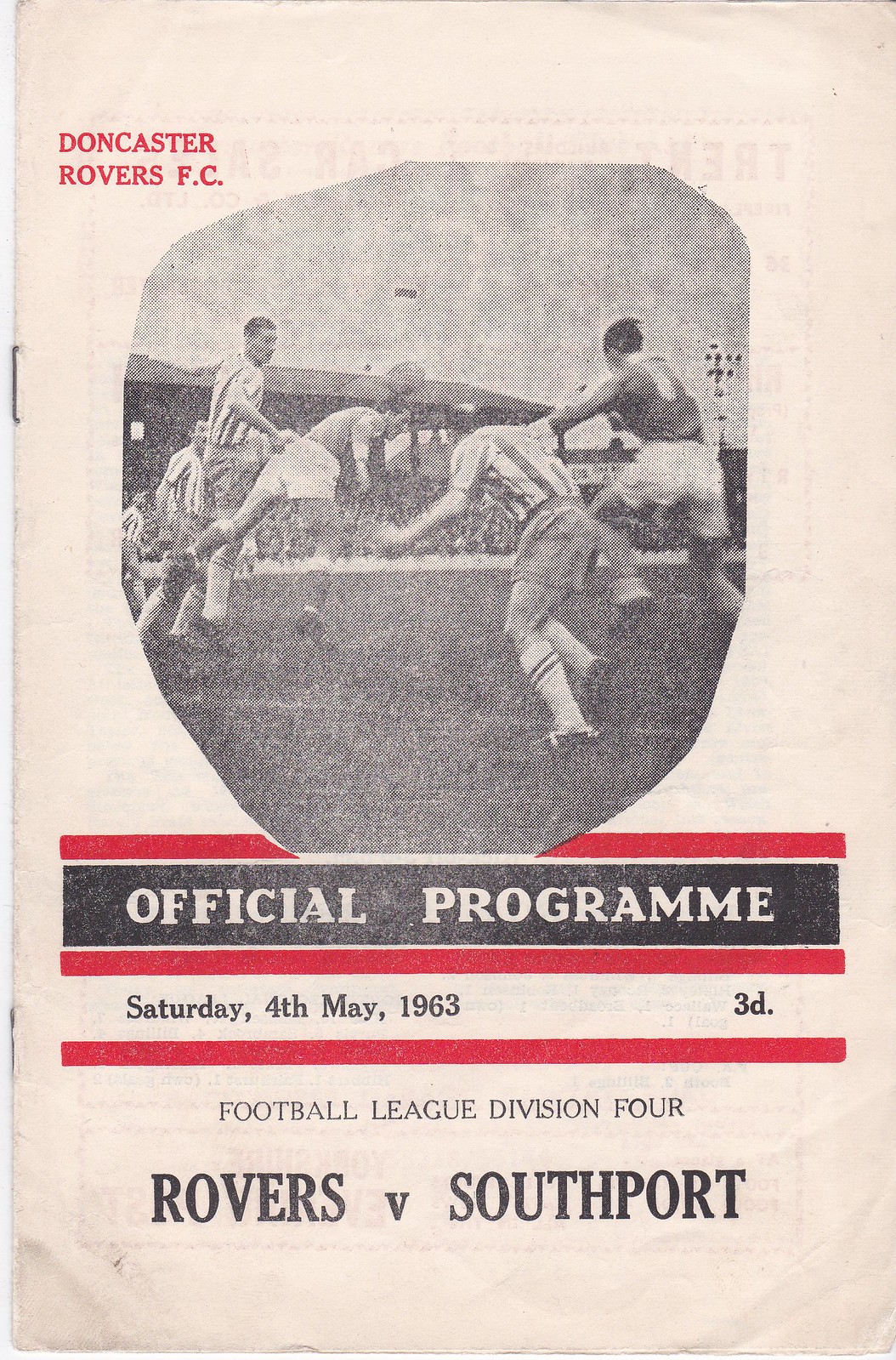The image is the front cover of an old sports program booklet, specifically for a football (soccer) match. The cover features a photograph at the top, showing several players on a field, wearing various football uniforms, seemingly engaged in play. In the sky above them, referees are depicted. The photograph is in black and white, contrasting with the aged, textured paper of the program which is tan in color, showing signs of wear and age.

At the top of the program, prominently in red text, it reads "Doncaster Rovers FC." Below the photograph, additional details are provided in various fonts and colors: "Official Program" is set within a black rectangle in light tan lettering. Further down, important match details are listed: "Saturday, 4th May, 1963, 3D," followed by "Football League Division IV," and in large print at the bottom, "Rovers vs. Southport." The alignment of the text places most of the information towards the bottom of the cover. Overall, the design and styling of this program suggest it's an authentic piece used by spectators attending a football match in 1963.